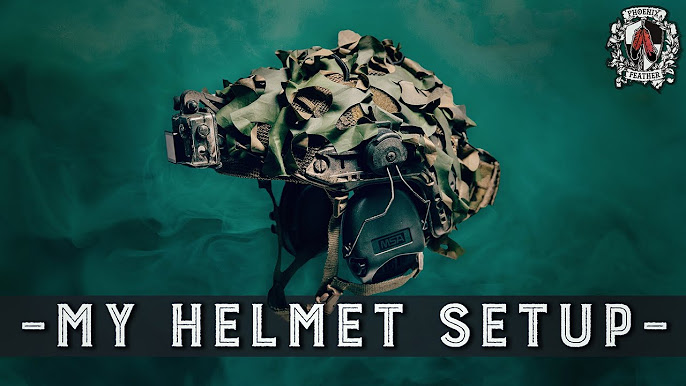The image showcases a soldier's helmet prominently positioned in the center against a green backdrop, reminiscent of leaves or green smoke. The helmet, rendered in camouflaging shades of brown and green, features a small, cubic light-emitting device on its front, likely used for tactical purposes. On the left side of the helmet, there are green-colored headphones emblazoned with the text "MSA." Below the helmet, engraved in white ink with black lines running through each letter, is the title, "My Helmet Setup," set against a black rectangular background. In the top right corner, there is a distinctive logo reading "Phoenix Feathers," depicting two red feathers with black tips inscribed within a white and black shield.